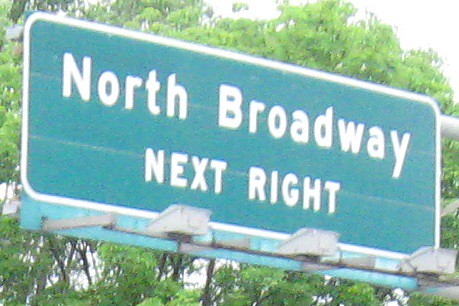The photograph captures a daytime scene with a somewhat grainy quality. It features an overhead street sign that reads "North Broadway, Next Exit." The sign is green with white text, enclosed within a white rectangular border. Below the sign, there are boxy white-colored lights visible. In the background, an array of trees fills the scene, showcasing lush, thick green leaves in varying shades from light to dark. The upper part of the image has some light glare. Behind the sign, bare brown tree branches are also visible. The sign shows signs of age and distress, with noticeable discoloration and lines running through it, as well as corrosion at the bottom.